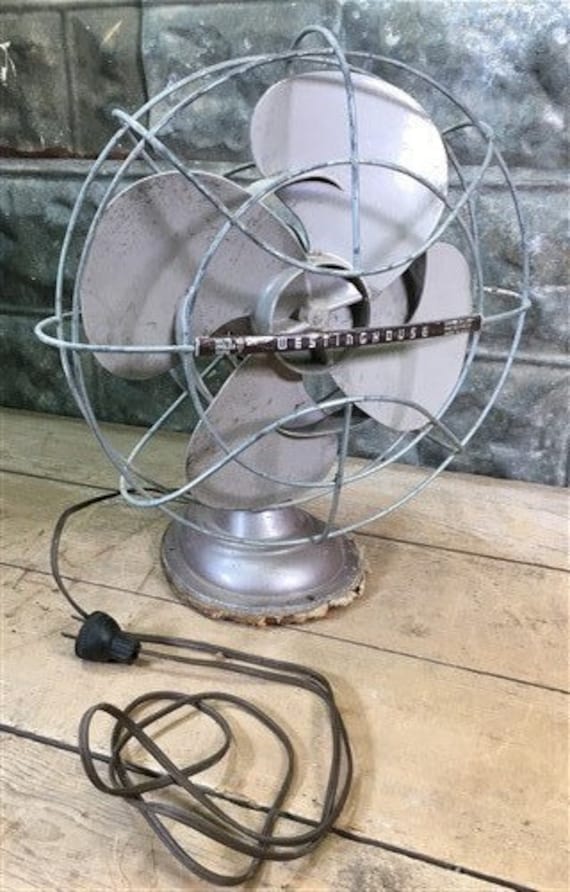This close-up photograph features a vintage Westinghouse desk fan, likely from the 1930s or 1940s. The fan, constructed entirely of silver metal, showcases a simplistic yet functional design. Encased in a wiry cage, its thick silver blades hint at a bygone era of craftsmanship. The front of the fan prominently displays the "Westinghouse" brand name across one of its metal bars. The fan’s base shows tarnishing around the edges, adding to its aged appearance. A coiled black cord emerges from the back, leading to a dated plug that further emphasizes the fan’s historical value. The fan sits atop a light-colored wooden plank table, its rustic charm complemented by a backdrop of a gray, bumpy stone wall composed of multiple uneven stones, adding texture and character to the scene. The overall distressed state of the fan underscores its long-term use and durability.